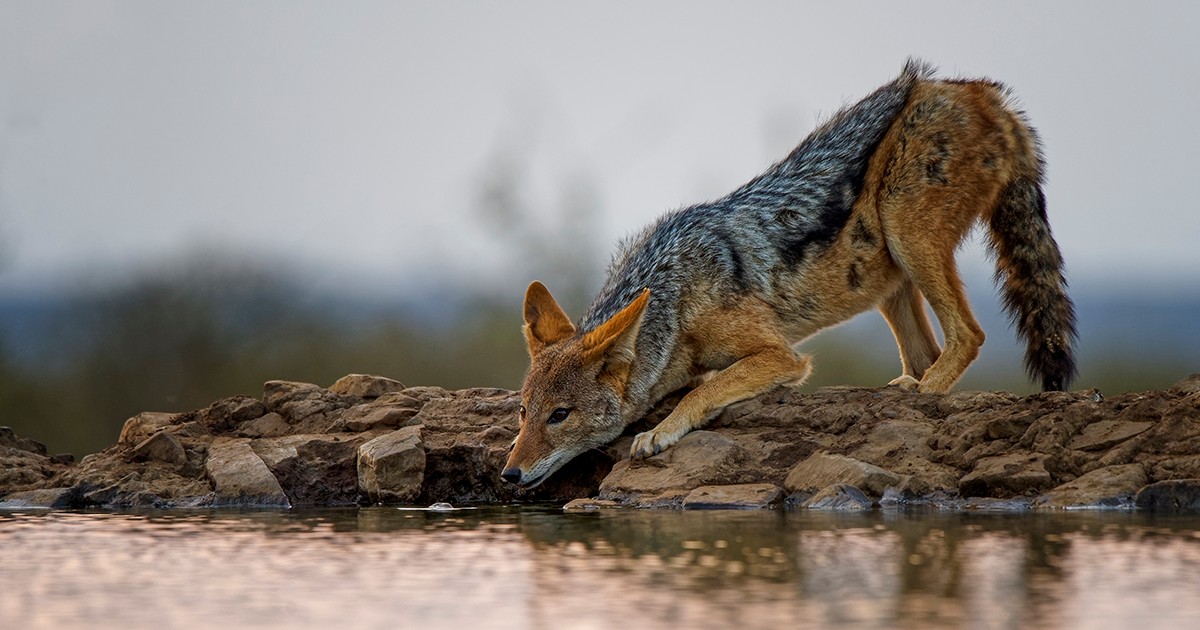A professional nature photograph captures a striking scene of a wild canid—likely a wolf—poised gracefully on the edge of a rocky pond, intently gazing into the water as if preparing to take a sip or hunt a water creature. The wolf's richly colored coat features a gradient of grays on its top, transitioning into shades of ginger and brown on its legs, head, and tail. This marked change in fur coloration perhaps suggests the shedding of a winter coat, giving way to a summer coat. Its black nose hovers just inches above the water's surface, which is dotted with small bubbles, enhancing the suspense of the moment.

The wolf's body is in a crouched position, front legs bent and ears erect, embodying a sense of focus and alertness. The surrounding environment, though artfully blurred in the background, hints at a serene natural setting that includes rugged mountains and dense foliage under a sky that frames the scene beautifully. This expert use of depth of field ensures the viewer's attention remains fixed on the wolf’s concentrated demeanor and intricate fur details, which include patches of white around its mouth and along the top of its back. The tan-colored rocks underfoot contrast subtly with the reflective waters of the lake, completing this immersive wildlife depiction.